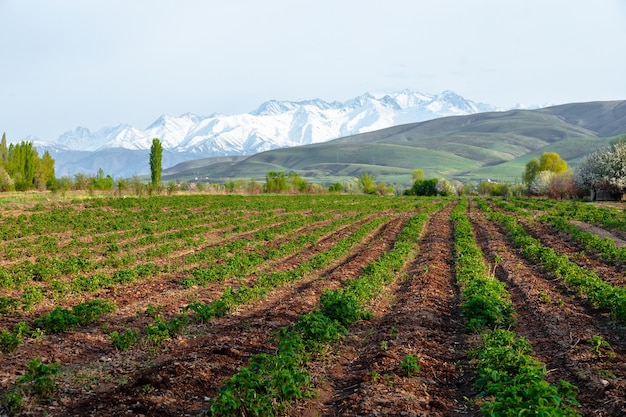This photograph captures a serene rural scene that stretches out into the distance. In the foreground, meticulously neat rows of small green plants signal the early stages of the growing season, emerging from rich brown soil. The symmetry of the rows is broken only by the occasional bit of dirt visible between them. As you move further back in the image, the middle ground reveals trees in full leaf, interspersed with a few neatly manicured and wide deciduous trees. The hills transition from lush green to light brown, creating a layered backdrop against the grand vista beyond. Dominating the horizon are majestic snow-capped mountains, resembling ranges such as the Cascades or the Rockies, under a pale gray sky. The entire scene is bathed in the glow of a bright sunny day, evoking a sense of tranquility and the barrenness of human presence, with nature flourishing in its untouched state.